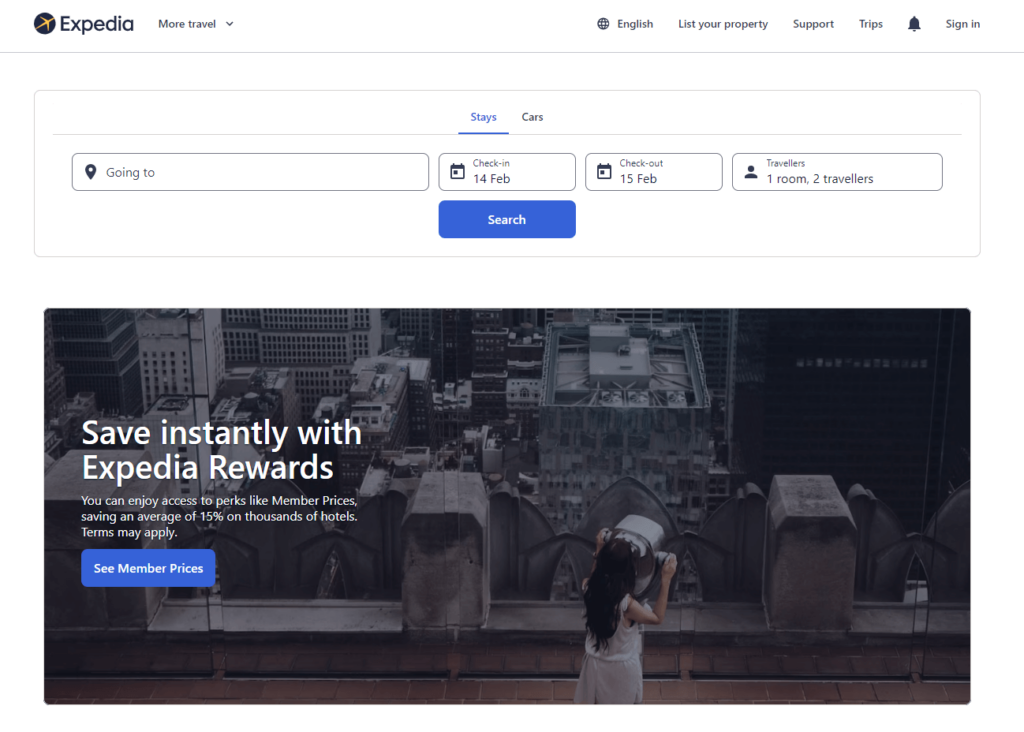This image depicts the Expedia website's user interface. On the left side, the words "More Travel" are prominently displayed. Several navigation tabs are located beneath this, including options for selecting the language (currently English), listing your property, accessing customer support, viewing your trips, and notifications indicated by a bell icon, followed by a sign-in option.

Central to the image is a search box with various options. The top bar allows users to choose between "Stays" and "Cars." Below, the fields for entering details appear: a text box for the destination, and date fields showing check-in on February 14th and check-out on February 15th. The travelers' field indicates one room for two travelers. A prominently placed "Search" button is situated to the right of these fields.

An eye-catching, grayed-out background image features a young girl peering through binoculars from the top of a building. Overlaying the right side of the image is a promotional text stating, "Save instantly with Expedia Rewards," emphasizing the benefits of membership such as access to exclusive prices and perks.